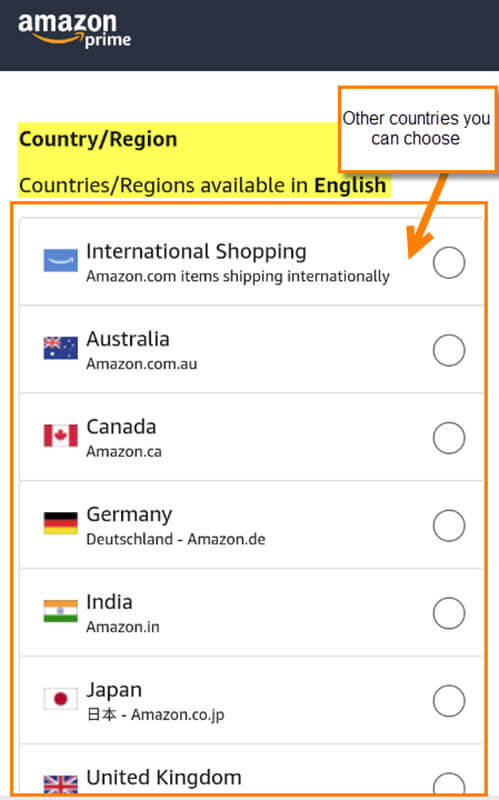The image displays a screenshot of a mobile device showcasing the Amazon Prime shopping app. At the top of the screen, there is a black horizontal banner featuring the Amazon Prime logo in white, with the iconic yellow curved arrow beneath the word "Amazon". Directly below the banner, a highlighted yellow section reads "Country/Region". Underneath this, it specifies "Countries/Regions available in English". The main section of the screen displays a list of different countries. Prominently, there is an orange rectangle containing a black text that states "Other countries you can choose", accompanied by an orange arrow pointing towards "International Shopping" and "Amazon.com, items shipping internationally". This image provides a detailed view of the options available for international users to select their country or region for Amazon Prime services.